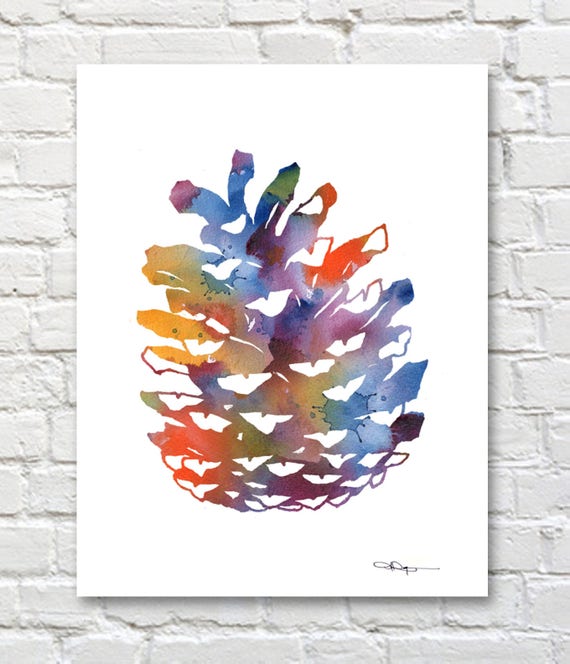In the image, a painting of a pine cone, done in vibrant watercolors, is mounted on a white piece of paper against a uniformly painted white brick wall with 13 visible rows of bricks. The pine cone is depicted with layers, akin to an actual pine cone, but instead of natural colors, it features a spectrum of rainbow hues including purple, red, yellow, blue, green, and orange. The colors blend together in an ombre effect and are segmented by white outlines, highlighting the structure of the pine cone. The painting's base starts at the bottom right, angled upwards towards the top left of the image. There is an illegible autograph in black ink at the bottom right corner of the paper. The paper is perfectly centered both horizontally and vertically against the white brick backdrop, emphasizing the detailed and colorful representation of the pine cone.